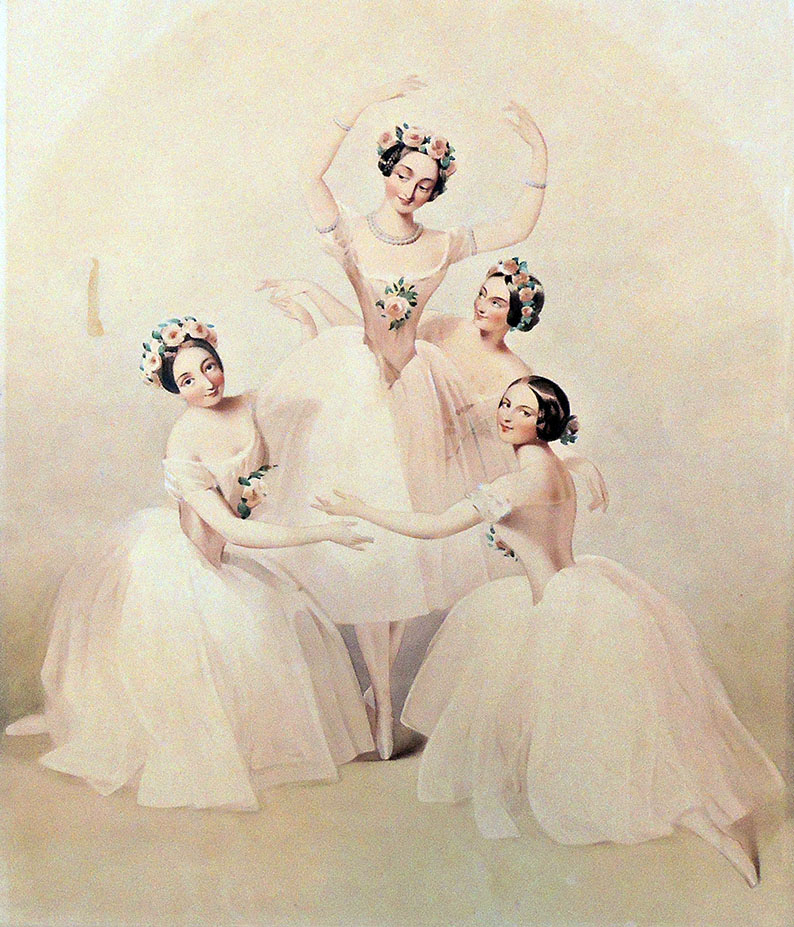The image illustrates a captivating scene of four ballerinas, all with dark hair styled in buns adorned with headbands of pink flowers and green leaves. Central to the composition is a ballerina standing gracefully on her tiptoes, her arms elegantly raised above her head in a classic ballet pose. She dons a skin-tight pink bodice and a voluminous tutu that extends just past her knees, accentuated by a pink flower on her chest. Surrounding her are three other ballerinas, each kneeling at her waist, creating a circle around her. They are dressed similarly, in matching pink tutus and bodices, each accessorized with floral headbands, except for one who has no flowers in her hair. The background of the painting is a light tan color, adding a soft contrast to the delicate hues of the ballerinas' outfits and the floral adornments. Their poses and interconnected arms suggest a harmonious and intimate ballet routine, capturing the elegance and grace of their performance.